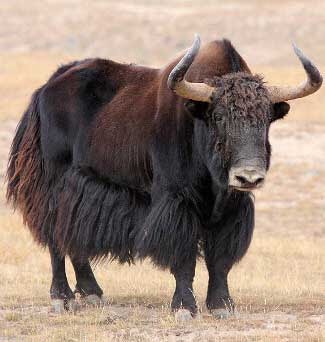This color photograph captures a large yak standing on a field of dead brown and yellow grass. The yak features long, sharply pointed horns that curve upward like those of a Texas longhorn steer. Between the horns, a dark brown, shaggy tuft of hair crowns its head, which is predominantly almost black, save for some white fur around its dark eyes and nose. The yak's muscular frame is notable, with a prominent hump or withers just behind its head covered in lighter brownish-orange fur that extends down its back. The area beneath its belly and along its legs is adorned with long, shaggy, and curly black fur, contrasting against the cropped appearance of the rest of its coat. Near the tail and hind legs, the fur takes on a more reddish-orange hue, remaining long and wiry. The yak stands imposingly, gazing directly at the viewer, its impressive stature and rich, varied coat making it a striking presence in the photograph.